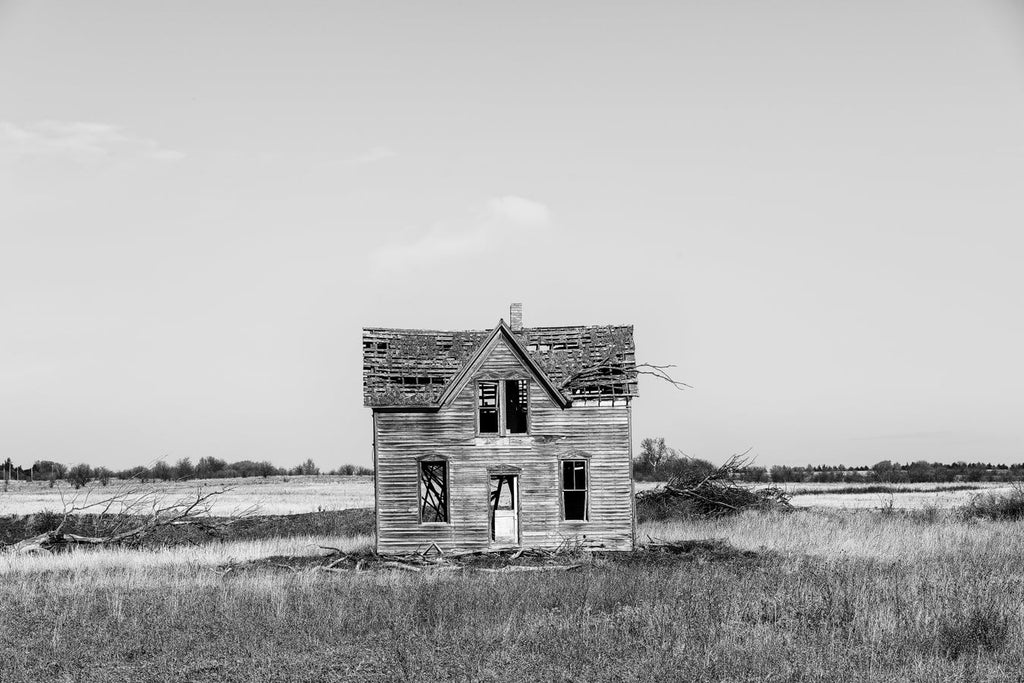This black and white photo captures a small, two-story wooden house standing solitary in a grassy, largely barren field, likely a prairie. The house is clearly dilapidated, with a roof in severe disrepair—several shingles are missing, creating gaping holes. Parts of the roof have completely fallen apart, and broken tiles are scattered about. You can see through the frame in some areas, emphasizing its neglected state. The house features a front door, located between two windows on the ground floor, with another window directly above the door on the second floor, along with a chimney. Strikingly, tree branches protrude from both sides of the rooftop, suggesting recent storm damage, possibly from a tornado. The windows are broken, the door frame stands open, and a large hole in the back of the house is visible through one of the front windows, partially covered by vines. The grass surrounding the house is tall, with only a few trees visible in the distant background, highlighting the isolation and abandonment of this early 1900s structure.